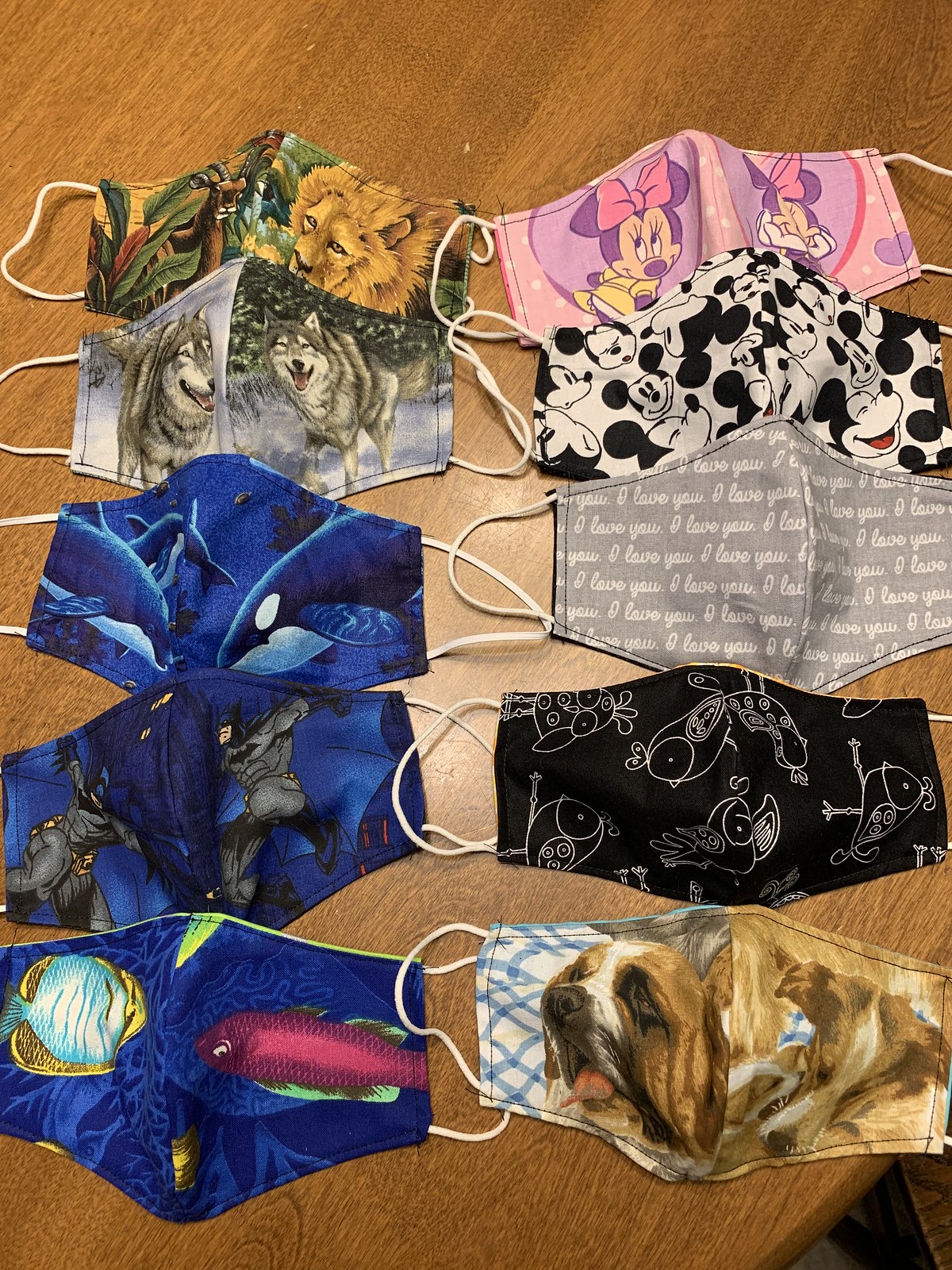This photograph features ten cloth face masks, commonly used during the COVID-19 pandemic, displayed on an oval, wooden table. The masks are arranged in two neat columns of five, laid out in a portrait orientation. Each mask boasts a unique design and vibrant colors:

- The top left mask showcases a jungle theme with green leaves and a lion.
- Beneath it is a mask adorned with two wolves, their bluish-white snouts contrasting against a background of trees.
- The third mask on the left features three killer whales set against a dark blue backdrop.
- Following that is a mask with a Batman theme, also on a dark blue background.
- The last mask in the left column depicts two fish with a jellyfish pattern in the dark background.

In the right column:
- The top mask is pink and purple, featuring Minnie Mouse.
- Below it is a black and white mask with Mickey Mouse.
- The third mask has the phrase "I love you" repeatedly printed in white cursive on a gray background.
- The fourth mask is black and white, decorated with a whimsical pattern, possibly birds or cartoony fish.
- The final mask in the bottom right corner portrays a sad-looking dog, resembling a St. Bernard, with a brown and white coat, black nose, and eyes.